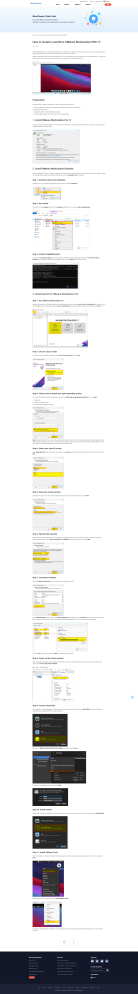The image showcases a densely detailed webpage displayed on a desktop computer. The header features a prominent blue box with some writing, emphasizing it as an important or clickable element. Below this, the navigation bar contains four distinct black tabs and is accompanied by a striking red button on the right side, likely a call-to-action.

Central to the webpage, there is a distinctive oval-shaped or donut-like blue image, surrounded by various colorful boxes that seem to orbit it, suggesting interactive elements or related information. On the left, there is a black heading, although its content is illegible. Below it, another black title and a paragraph of standard, non-bolded text provide additional information.

Midway down the page, there is a stretched-out image resembling a smartphone, with clickable icons or Google images beneath it. This section is introduced by a bolded title followed by descriptive text.

Further down, a dialog box with accompanying text appears, framed by another black title and description. A highlighted segment, possibly a demonstration of how to interact with a document, stands out in yellow. This is flanked by a few more images displaying similar procedures.

The bottom section features a black screen with visible script, assorted boxes in predominantly white and some black, concluding the image composition.